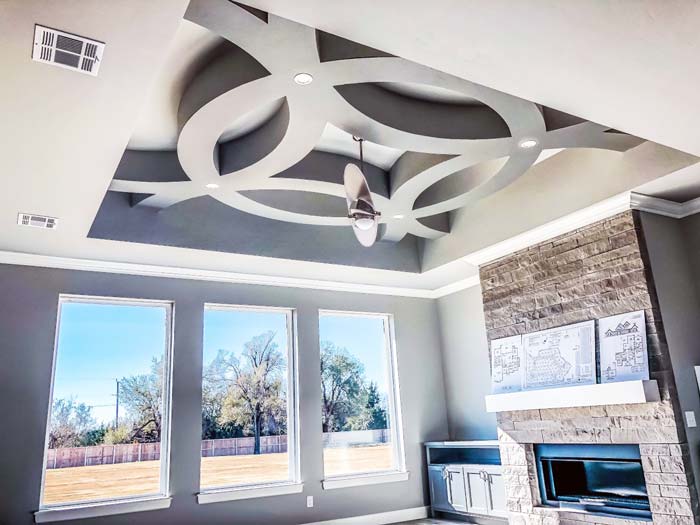This image captures an elegantly-decorated living room, showcasing its upscale and meticulous design. The left side of the room features a grey wall punctuated with three large vertical rectangular windows, allowing ample natural light to pour in and providing a scenic view of a vast beige grass field bordered by a wooden fence, with a backdrop of tall trees. Adjacent to this wall is a striking stone fireplace with a grey stone façade and a grey mantel adorned with what appear to be maps. To the left of the fireplace sits a grey wooden chest with two sets of doors and a shelf above. 

The room boasts a tall, intricately designed ceiling, painted a light grey, with a recessed square housing a complex circular pattern and semi-circles that resemble a pound sign. From the center of this pattern hangs a chandelier, surrounded by four white lights. The room's walls are painted grey, contrasting beautifully with the cream-colored ceiling. The overall aesthetic suggests that this is part of an upscale home, possibly a subdivision home or mansion, with its meticulous design elements and high-end finishes.